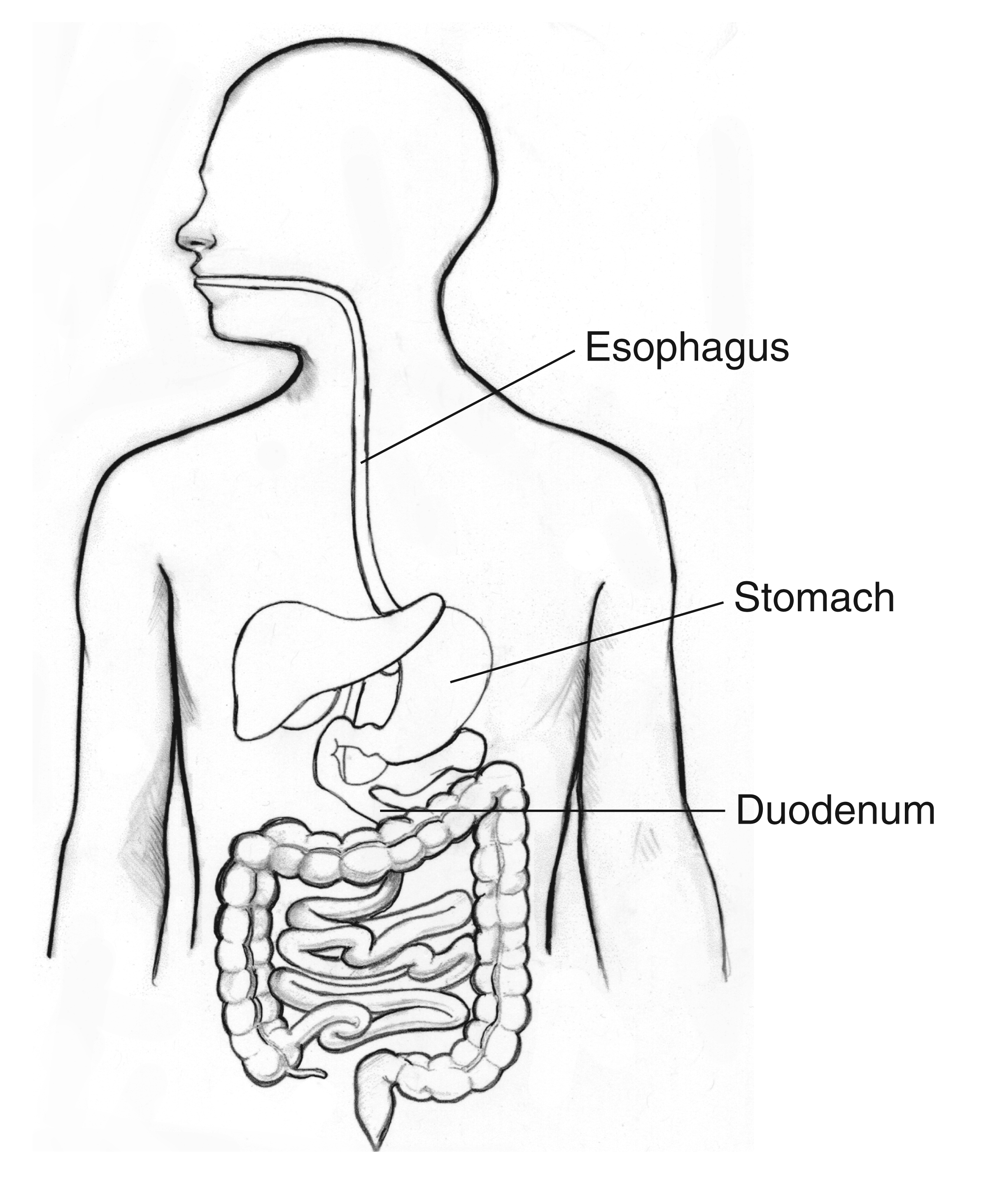This black ink diagram depicts the major parts of the human digestive tract within the outline of a man shown from head to waist, with his head oriented to the left, revealing the internal structure. The image primarily focuses on the digestive system, excluding the heart and lungs to highlight the relevant organs. The tract begins with a tube, starting from the lips, labeled "esophagus," extending down to the stomach. Below the stomach, a label points to the "duodenum," a section connecting the stomach to the intestines. The diagram also includes detailed sketches of both the small and large intestines, providing a comprehensive view of the digestive system.